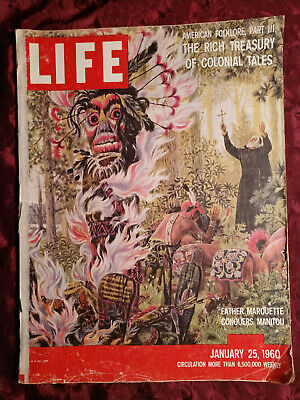The cover of the January 25, 1960, issue of Life magazine prominently features a painted image conveying a scene of colonial encounter. The top left of the cover showcases the iconic Life logo in bold white letters on a red background. In the top right corner, white text announces "American Folklore Part Three: The Rich Treasury of Colonial Tales." The illustration depicts a forest setting where a religious figure, possibly a priest or nun, dressed in black robes and a white headcloth, holds up a small golden cross with both arms raised. In front of this figure, several indigenous people appear to be kneeling or bowing, perhaps in prayer or submission. To the left is a striking large indigenous mask adorned with extensive feathers. The bottom right of the cover is dated January 25, 1960, with a caption reading, "Father Marquette Conquers Manitou," highlighting the historical context of the scene.